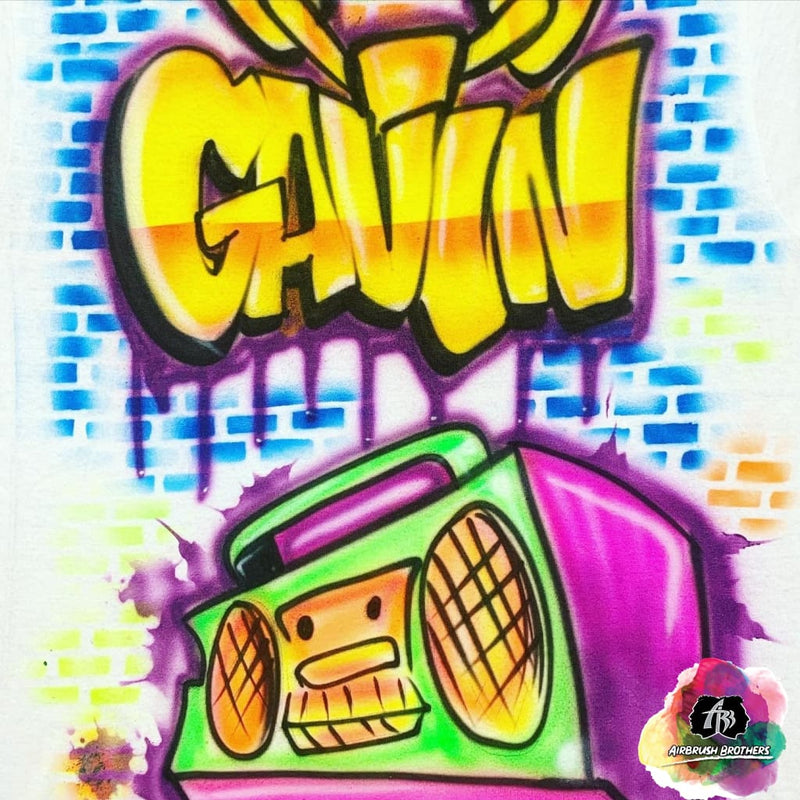This vibrant graffiti artwork features the name "Gavin" prominently displayed in bold, yellow bubble letters outlined in purple, set against a blue brick background with splashes of orange and yellow. The design exudes a cartoonish vibe, with "Gavin" seemingly suspended like a door knocker or necklace. Below the name, a colorful boombox radiates energy with its vivid green, pink, and purple hues, and yellow-orange speakers that resemble a face. The entire scene is meticulously airbrushed to create a dynamic and eye-catching illustration. In the lower right-hand corner, a small logo that reads "Airbrush Brothers" anchors the composition, adding a touch of authenticity and artistic branding to the piece.